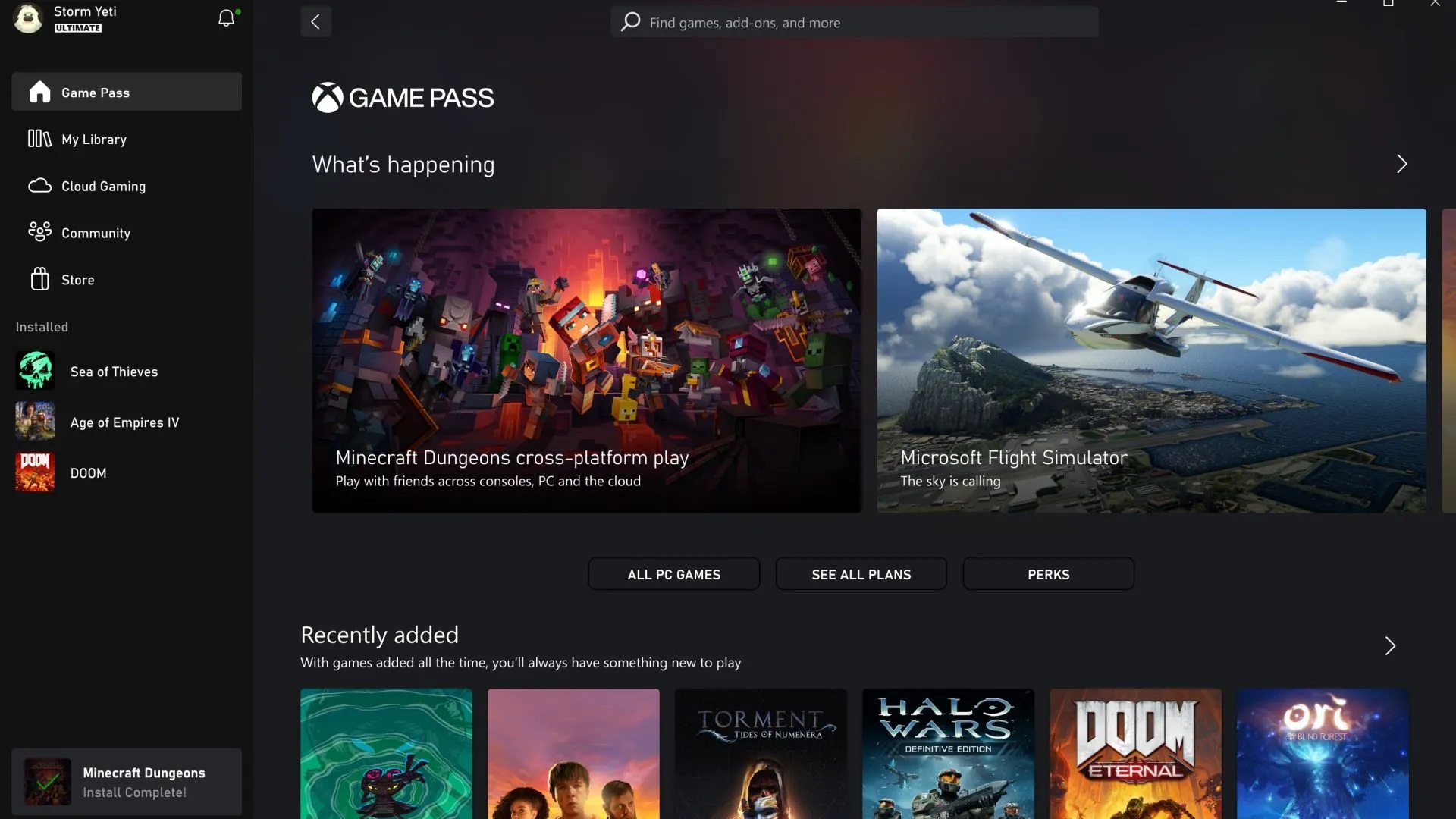The image portrays a vibrant entertainment website focused on PC and video games. The user is logged in under the username "Storm Yeti," with an avatar featuring a Yeti. The screen is divided into navigation sections on the left, including Game Pass, My Library, Cloud Gaming, Community, Store, and Installed. 

Within the Installed category, games such as Sea of Thieves, Age of Empires IV, and Doom are listed as installed. The Game Pass section is actively selected, showcasing the Game Pass logo and detailing current features. Among these are a Minecraft screenshot promoting cross-platform play in Minecraft Dungeons, and another from Microsoft Flight Simulator with the tagline "the sky is falling." 

Below these highlights, there are three interaction buttons labeled All PC Games, See All Plans, and Perks. The interface has a layout reminiscent of Netflix, featuring a "Recently Added" section that ensures users always have fresh games to play. This section displays the cover art of the newly added games, offering a visually appealing and user-friendly experience.